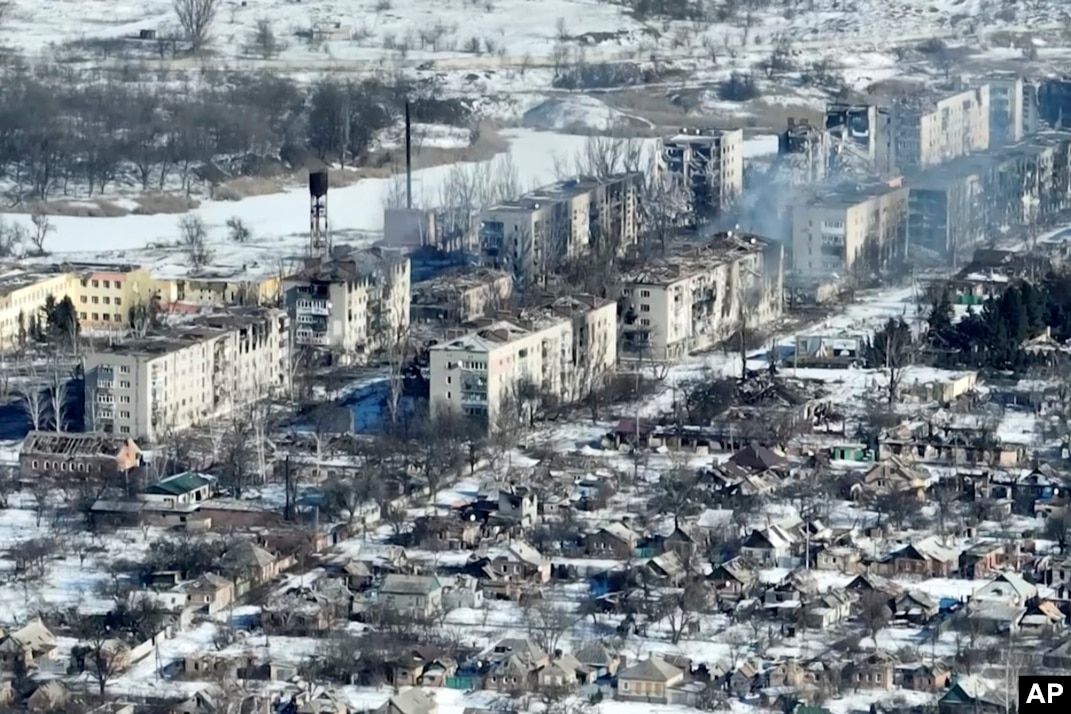The aerial image captures a small town blanketed in snow, divided neatly into a grid of residential buildings in the foreground and larger apartment buildings in the background. The town, possibly rural or industrial, seems to have experienced significant destruction, with many buildings in the background appearing half torn apart as if by an explosion. A distinct haze hovers over several areas, accentuating the somber scene. Structures like power lines and a water tower are visible near the left and back of the town. The presence of a black box with white "AP" text in the bottom right hints at the Associated Press's involvement. The photograph's landscape and architecture suggest it could be a depiction of a post-disaster site, possibly somewhere like Russia.